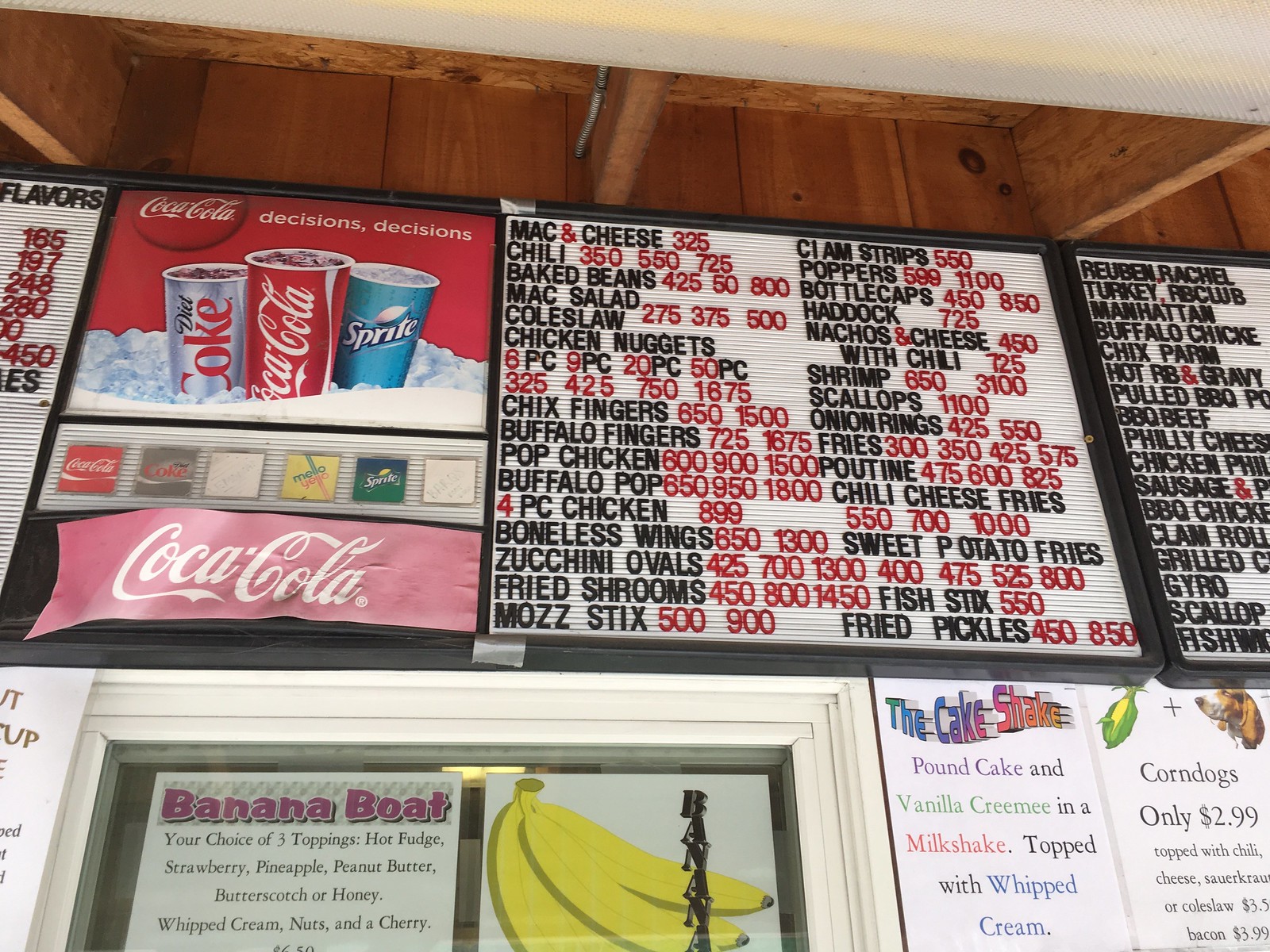The image depicts an outdoor takeout station adorned with a series of detailed menus positioned above the serving window. Dominating the scene is a Coca-Cola advertisement, featuring three large soft drink illustrations along with their respective names and a tile icon below each. The banner, matching the dimensions of the nearby menus, is mounted directly above the food-serving window.

To the right of the Coca-Cola advertisement is an extensive menu listing various American food items. The items are written in black text, with prices highlighted in red for easy visibility. Adjacent to this is another menu, styled similarly, but partially cropped, making some details unreadable.